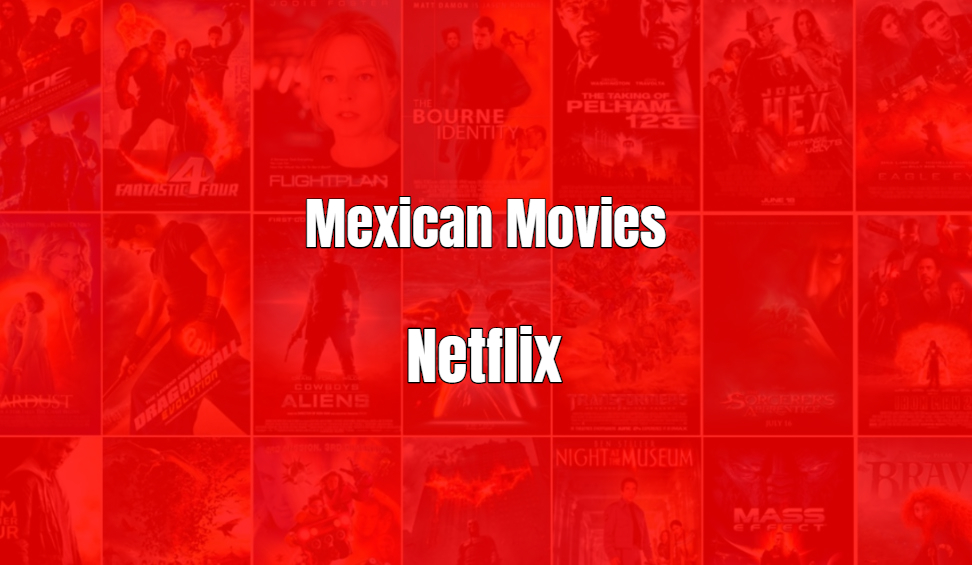The image is a horizontal rectangle resembling a Netflix webpage, predominantly colored in red with orange and brown hues. The focal point is the large white text in the center that reads "Mexican movies" with "Netflix" right below it. Overlaid with a translucent red film, the background displays about 21 movie covers which appear washed out and barely discernible. Among the few visible titles starting from the top, one can identify "Fantastic Four," "Flight Plan," "The Bourne Identity," "The Taking of Pelham 123," and "Jonah Hex." The middle section reveals "Dragon Ball: Evolution" and another poster hinting at an alien theme. Near the bottom, visible but somewhat cut off, are "Night at the Museum," "Mass Effect," "Brave," and "The Dark Knight." Overall, while the exact clarity of each movie cover is compromised due to the red overlay, the recognizable titles hint at a diverse range of films.